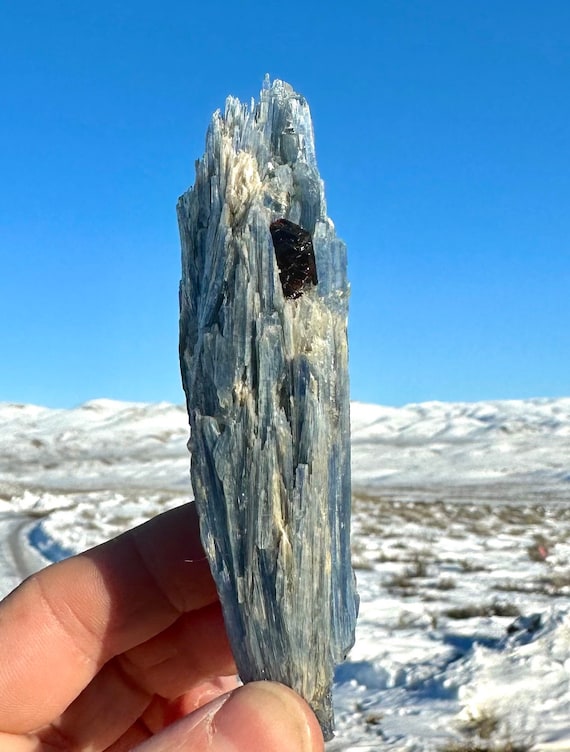A vertically rectangular photo captures a clear, sunny day with a bright blue, cloudless sky transitioning into a slightly darker blue towards the top. The foreground features a hand, partially visible from the bottom left corner, thumb and fingertips grasping a large, thin shard of a mineral-like rock, which is light blue-gray with sheets that appear almost transparent at the center. Embedded within this rock is a smaller, darker stone. The snowy landscape in the background is slightly out of focus, revealing a snow-covered field scattered with brown grass and a dirt road extending into the distance on the left. Further back, a snowy hillside stretches across the middle of the image, adding depth and emphasizing the cold, wintery setting.